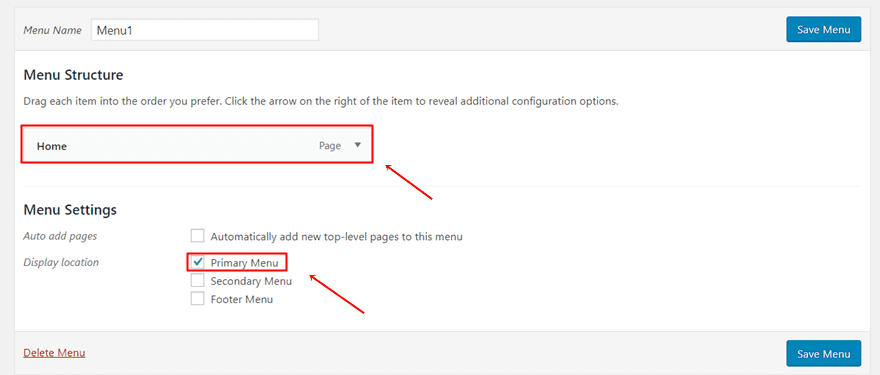The image displays a detailed chart with a structured interface. 

**Header Section:**
- The header has a light grey background.
- On the left-hand corner, there’s a text box labeled "Menu Name," which contains the text "Menu 1."
- On the far right, a prominent blue "Save Menu" button is visible.

**Main Body:**
- Below the header, the background shifts to white.
- On the far left, there is bold black text labeled "Menu Structure."
- In smaller text beneath this label, it instructs: "Drag each item into the order you prefer. Click the arrow on the right of the item to reveal additional configuration options."

**Menu Items:**
- There is a drop-down menu titled "Home," boxed in red.
- To the right of the "Home" menu item, it indicates "Page" with another drop-down menu labeled as "Page."
- A red arrow points from the bottom towards this "Page" section, emphasizing it.

**Menu Settings:**
- This section contains four checkboxes:
  1. "Automatically add new top-level pages to this menu"
  2. "Primary Menu" enclosed in a red box with a red arrow pointing from the bottom, indicating it is selected.
  3. "Secondary Menu"
  4. "Footer Menu."

**Footer:**
- At the bottom left corner, there's an underlined "Delete Menu" link.
- On the far right corner of the same row, there is another "Save Menu" button. 

The overall layout is clearly structured, with red boxes and arrows used to highlight essential elements.